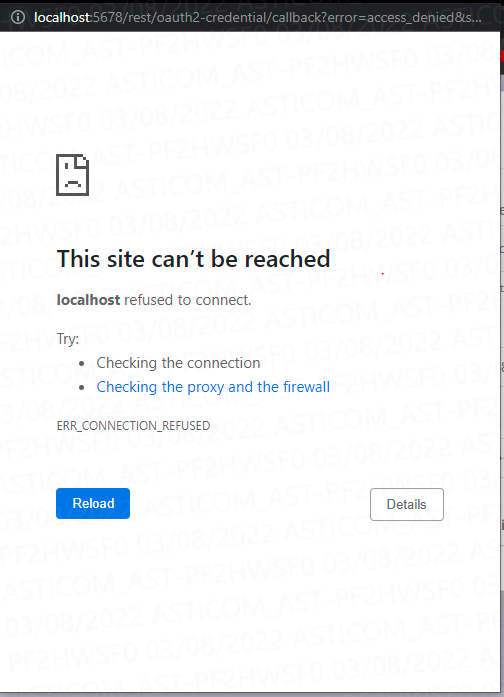This image is a watermarked screenshot of a non-functional website displayed in a web browser, notably Google Chrome. At the top of the screen, the address bar reveals that the website in question is being tested locally, as evidenced by the URL starting with "localhost:5678," followed by additional text related to the encountered error code. The browser is attempting to load a locally-developed site rather than a live one on the internet.

The error message is centrally featured and begins with a recognizable sad sheet of paper icon, indicating a loading issue. Directly beneath the icon, the text informs the user that "This site can't be reached," with "localhost" in bold typeface, stating that the connection was refused. A bulleted list suggests troubleshooting steps such as checking the connection, proxy, and firewall settings.

Further down, the specific error code is displayed: "ERR_CONNECTION_REFUSED." Below this message, two buttons are available for user interaction: "Reload," highlighted in blue, intended for retrying the connection, and "Details," bordered in light gray, likely offering more information about the error.